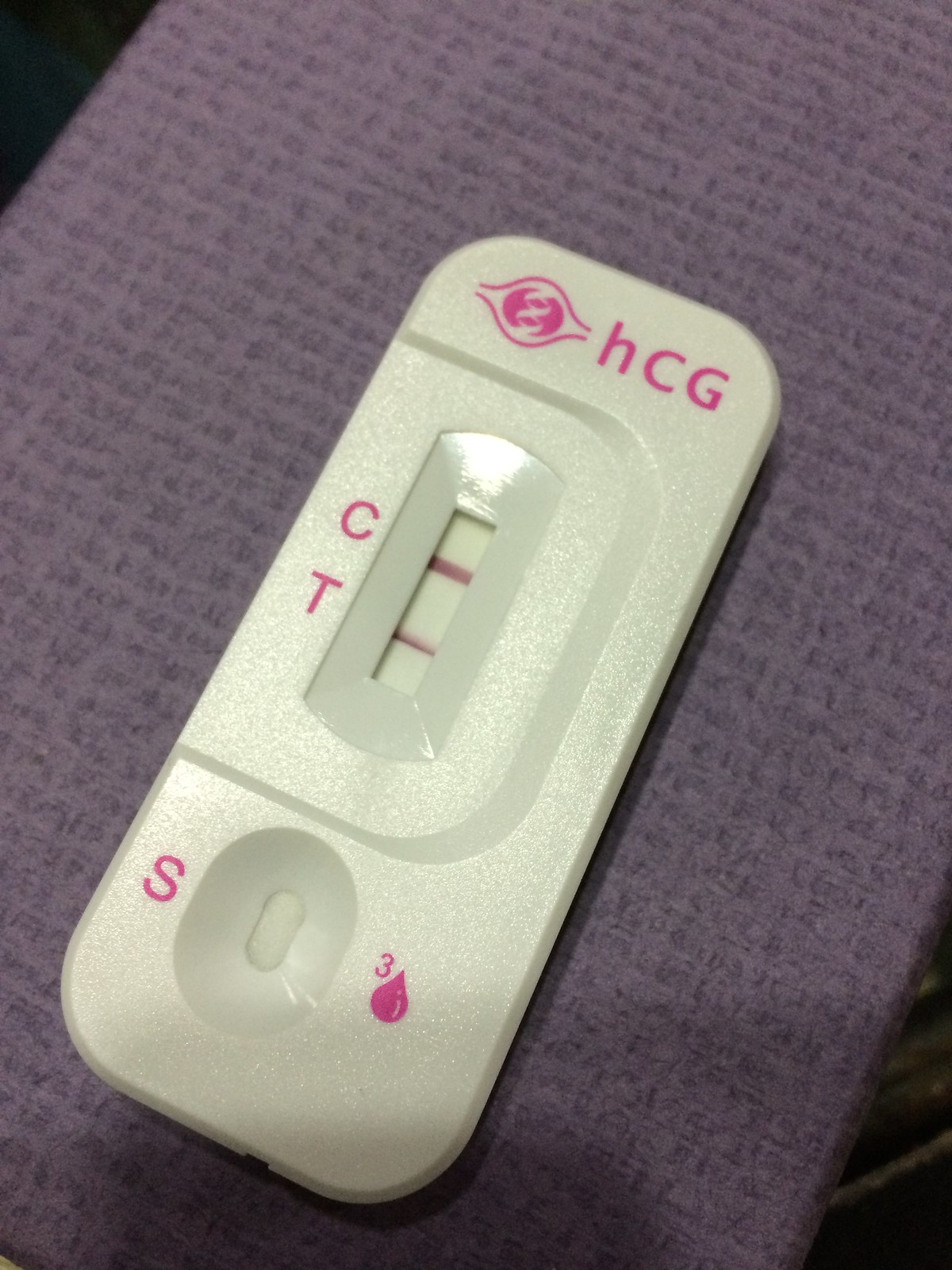This image features a close-up of a rectangular plastic medical test device, which closely resembles a pregnancy test. At the top of the device, there is a pink logo featuring a bulbous circle with a smaller circle inside, accompanied by the letters "HCG." Below the logo, an oval indention in the plastic encloses a small window displaying two horizontal pink lines, one adjacent to the letter "C" and the other next to the letter "T." 

Further down the device, another indention reveals a second window, which is unmarked but features a letter "S" to the left and a small number "3" with a teardrop icon to the right. The test rests on a purple background, which appears to be either paper or cloth, providing a contrasting backdrop for the white plastic device and its detailed inscriptions.